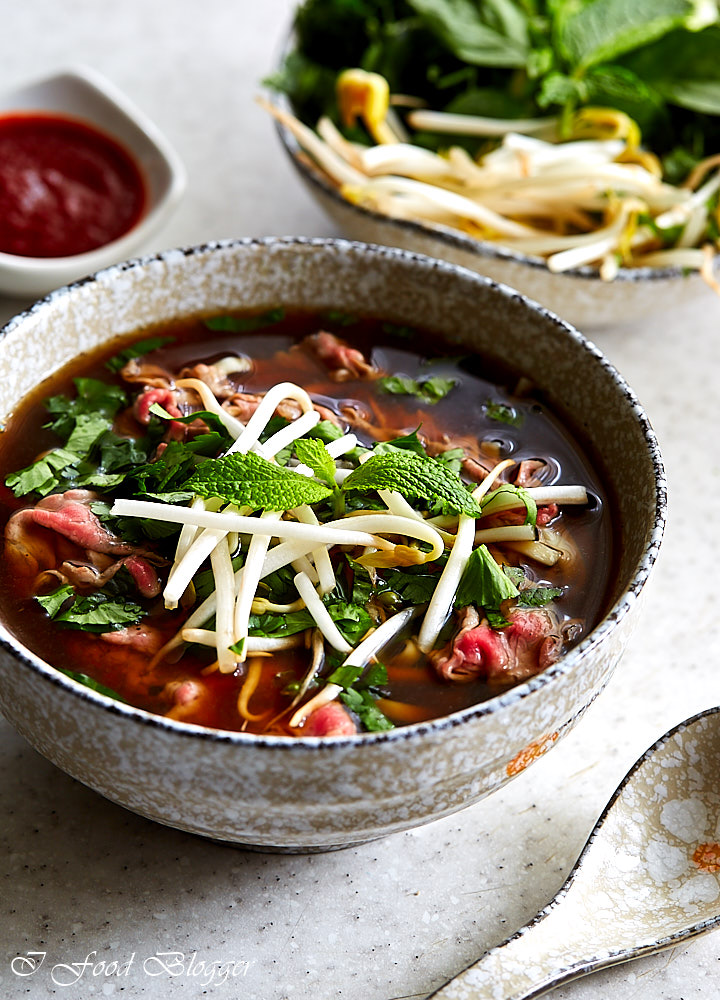The image showcases a tantalizing bowl of soup, likely a variant of ramen, nestled in a rustic, tannish clay bowl. The soup is a rich, brothy mixture, featuring visible noodles intertwined with vibrant green vegetables and succulent pieces of bacon. The hearty meal exudes warmth and depth, characteristic of traditional ramen dishes. Adjacent to the main bowl, on the left, is a small dish containing a red sauce, adding a contrasting burst of color and potential flavor enhancement. To the right of the main bowl is a similar clay bowl filled with the same soup, though this perspective does not reveal the brothy juices. At the bottom right of the image, a wooden spoon, closely matching the color and material of the bowls, rests on the table. The caption “A food blogger” is discreetly inscribed in white at the bottom left corner, identifying the source of this appetizing scene.